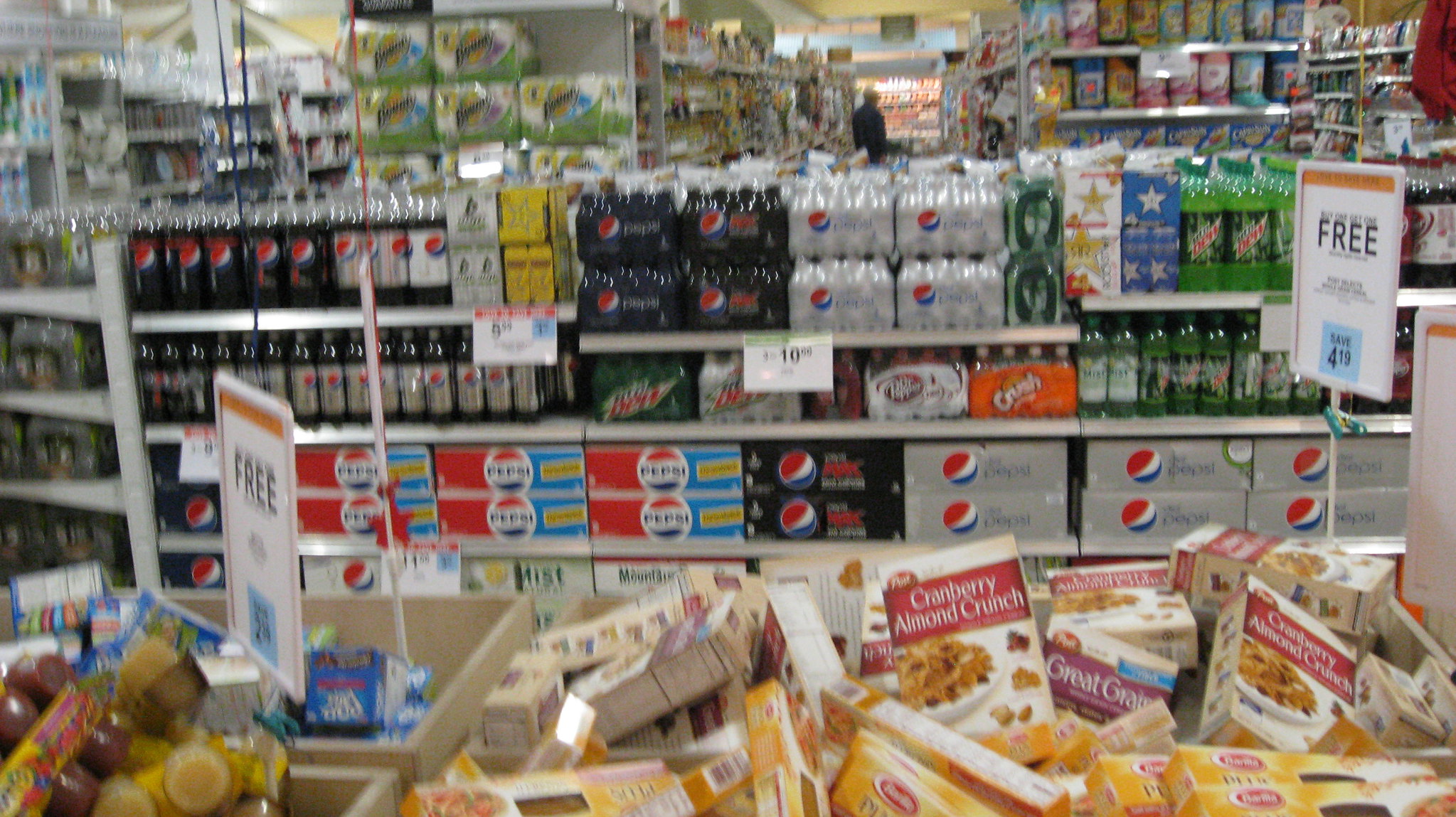In this vibrant image taken inside a bustling grocery store, the foreground is dominated by several bins brimming with assorted cereal boxes. Among the varieties visible are Cranberry Almond Crunch and Grape Greens, along with several other brands, all showcased enticingly in the bins. A prominent sign attached to the bins announces a tempting offer in bold letters, "Buy One, Get One Free," with an additional note in blue text stating, "Save for $4.19." 

Just beyond the cereal bins, several shelves are neatly stacked with a variety of soft drinks. The shelves display cases of Pepsi products, neatly arranged eight-pack bottles, and rows of two-liter bottles occupying the top shelf. White pricing signs, indicating the costs of these beverages, hang clearly from the shelves.

In the background, towering shelves laden with various food items stretch towards the ceiling. Amidst these shelves, a single shopper is observable, standing in one of the aisles. The individual, a taller person dressed in a black long-sleeve shirt, appears to be perusing the selections available, contributing to the dynamic and lively atmosphere of the grocery store scene.